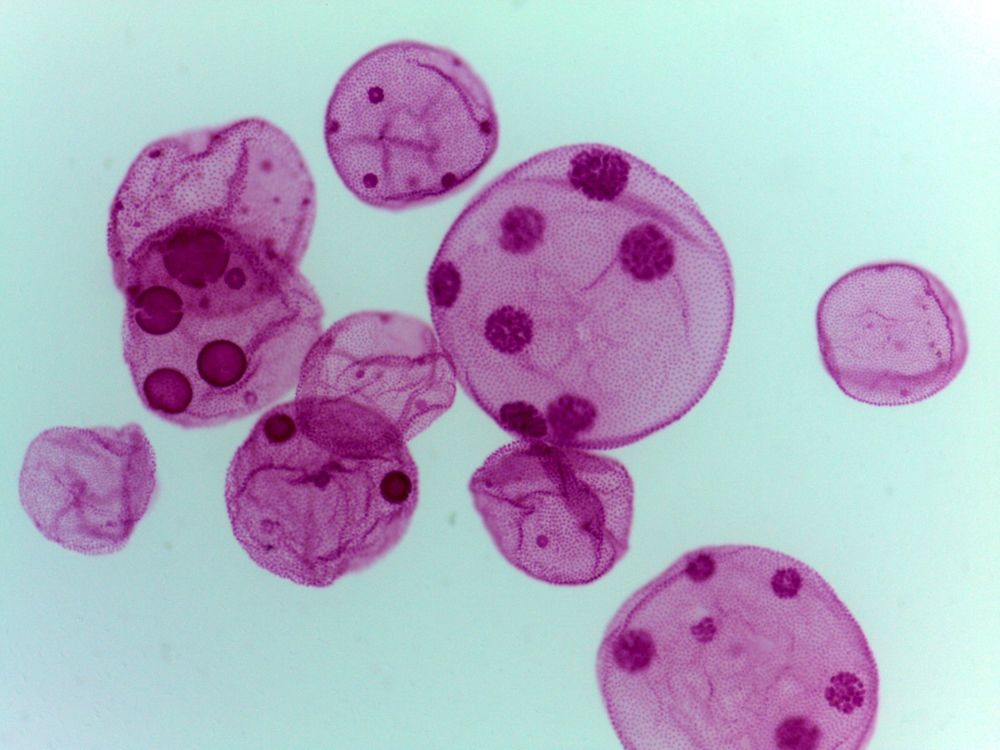The image depicts a cluster of purple, round structures with darker purple dots inside, set against a light blue-green background resembling sea foam. These circular shapes, some larger and others smaller, have a ridged edge and an overall translucent appearance, with occasional merging or touching. The structures resemble microscopic cells, possibly amoebas, with a jellyfish-like texture. Many of them are clustered towards the center-left, while a few, including a notably large one, are isolated on the bottom and center-right. The dark purple dots within these shapes vary in size and density, giving the impression of a textured surface. Overall, there are about eight or nine prominent shapes visible in the image.